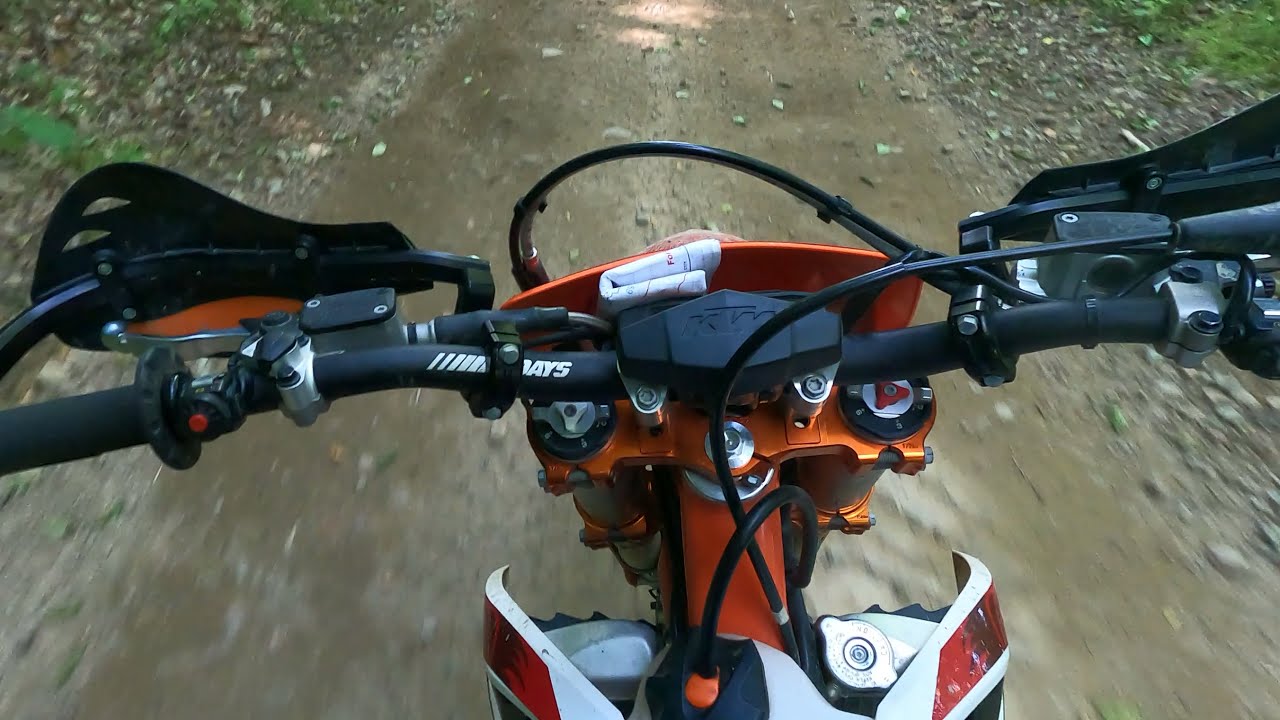This image captures a first-person perspective of a rider on an orange dirt bike, equipped with white and red accents on the body. The shot, likely taken with a GoPro, focuses on the bike’s handlebars, which are black with handguards for protection. Numerous wires and cables from the bike's brakes are visible, particularly on the top and middle sections. The handlebars also feature what appears to be writing or markings on the left side. The bike is traveling along a narrow dirt or gravel path, surrounded by rocks, and the trail is partially shaded with patches of sunlight filtering through. The handlebars have an orange shield, possibly containing a folded paper, and there is a radiator in front of the gas tank, typical for cooling purposes. The scene conveys a rugged, off-road adventure through a forested area.